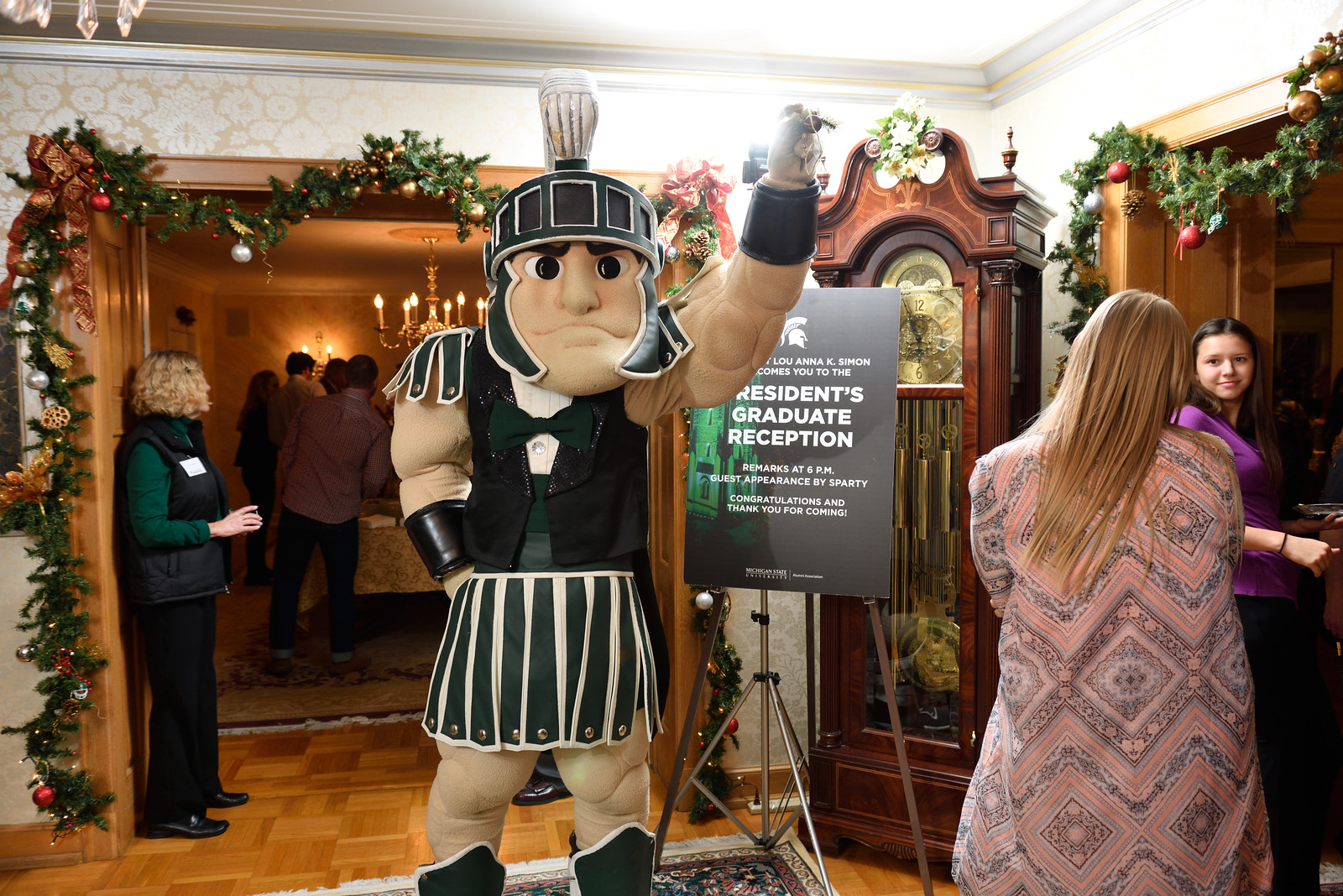Depicting a festive entrance to a school dinner hall, the image features doors adorned with Christmas-themed garlands and decorations. Centered prominently is a Spartan mascot, sporting a pleated skirt, helmet, and bow tie, symbolizing Michigan State University's spirit. The venue’s color palette includes green, black, beige, and grey, with grey floors grounding the scene. A significant feature is a grandfather clock positioned against the wall, accompanied by a welcoming sign that reads, "Louie Anna K. Simon welcomes you to the Residence Graduates' Reception, Remarks at 6 pm, Guest appearance by Sparty. Congratulations and thank you for coming."

To the right, two women are engaged in conversation as they approach a doorway, adding a dynamic element to the photograph. Meanwhile, on the left side, a single woman stands by another doorway, perhaps awaiting entrance. Behind these doorways, a banquet room can be glimpsed, highlighted by a large chandelier and matching wall sconces. The scene is lively and inviting, encapsulating the celebratory atmosphere of the graduates' reception.